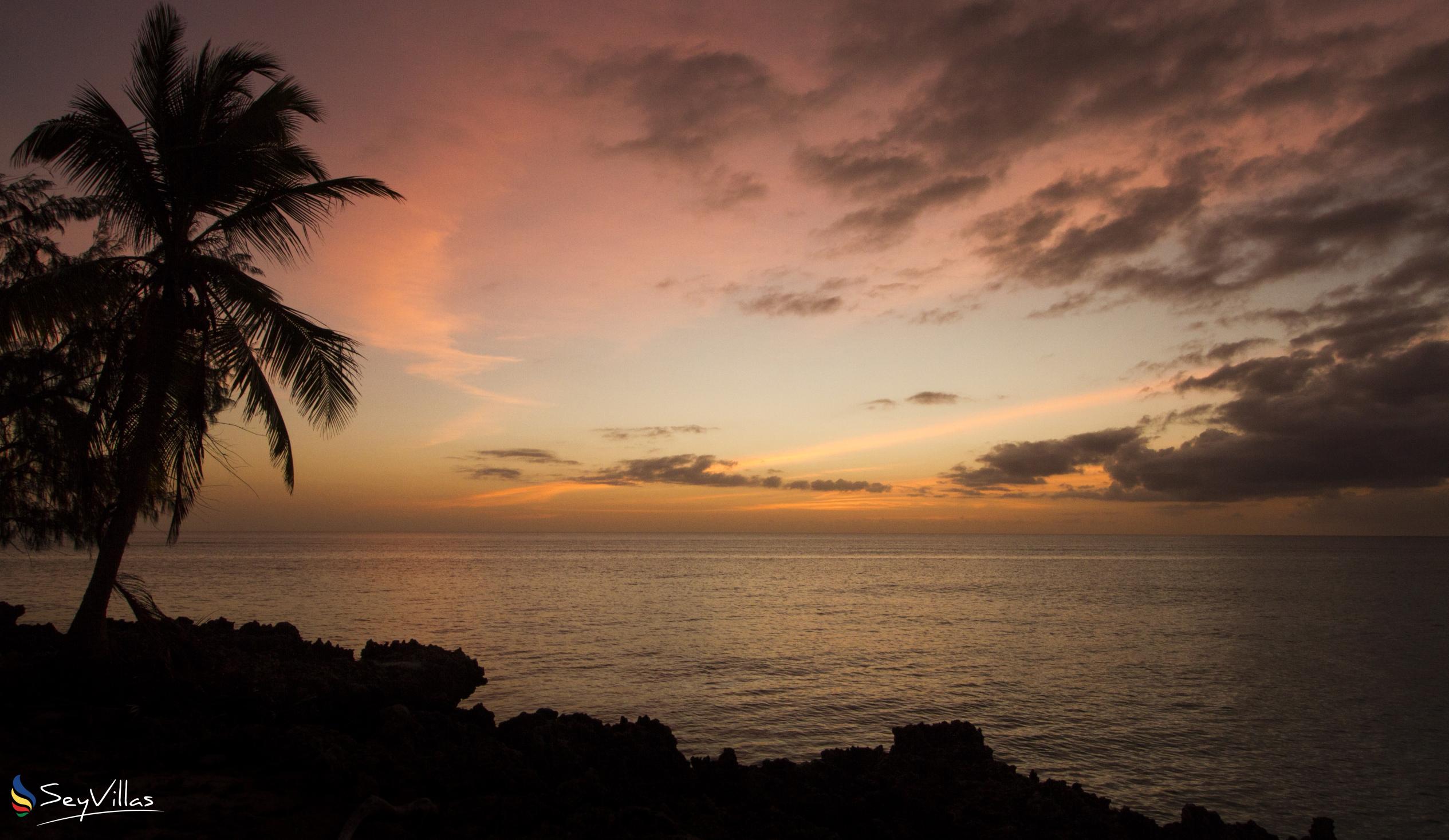The image depicts a tropical scene at what appears to be a place called St. Villus, indicated by white lettering near the bottom left of the image. A small, colorful flag – blue, yellow, and red – flutters next to this inscription. Dominating the left side of the frame are two palm trees; one leans inward toward the center of the image, while the other tilts outward. Below the palms, the foreground is covered in lush bushy terrain.

The ocean stretches across the middle and right side of the image, looking remarkably flat with no land in sight at the horizon. The sky above varies dramatically: the left side glows with shades of pink, indicating the low sun, while the upper right side is cloaked in dark, hovering clouds descending towards the horizon. Additional black clouds linger just above the horizon, emphasizing the approaching weather. The scene is a stunning juxtaposition of serene tropical beauty with the dramatic sky, further highlighted by the atmospheric conditions and the vivid hues of the twilight.